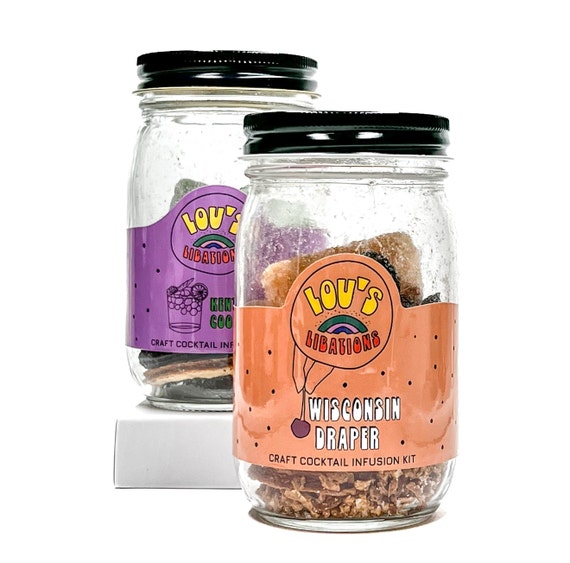This photograph features two glass bottles with black screw-top lids, prominently displaying the "Luz Libations" brand. The front bottle's label is orange with black dots, featuring a circular logo: "Luz" in yellow and "Libations" in red, with a dark green, pink, and purple three-stripe arc between the words. Below the logo, the label depicts two fingers pinching the stem of a cherry, accompanied by the words "Wisconsin Draper" in white, and the description "Craft Cocktail Infusion Kit" at the bottom. The bottle contains visible contents that appear to be spices or crushed nuts mostly obscured by the label. The bottle in the back has a purple label with the same "Luz Libations" logo. Beneath the logo is an illustration of a highball glass garnished with decorations. Both bottles are set against a plain white background, arranged with the orange-labeled bottle slightly in front, partially hiding the purple-labeled one, making the image ideal for e-commerce or retail display.